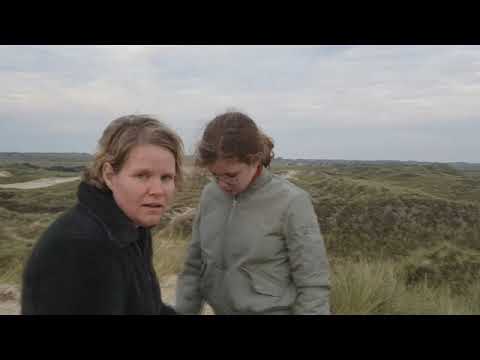In this outdoor daytime photograph, a Caucasian mother and her young daughter stand amidst a rolling, grassy field under a slightly cloudy sky. The mother, situated on the left side of the image, is seated and gazing directly at the camera, her mouth slightly open and expression neutral. She has blonde hair that drapes down both sides of her face and wears a black fleece jacket. Next to her stands the daughter, looking downwards at her lap, wearing glasses and a gray zip-up jacket that hints at a breeze. Both share similar blond hair, though the daughter's is tied back. The background reveals a picturesque landscape of greenish-beige, bumpy hills dotted with light green shrubbery and patches of sand. The image has a low resolution with noticeable compression artifacts and features horizontal black bars at the top and bottom, similar to widescreen movie frames. The color palette ranges from black and gray to light tan, dark green, off-white, and light blue.